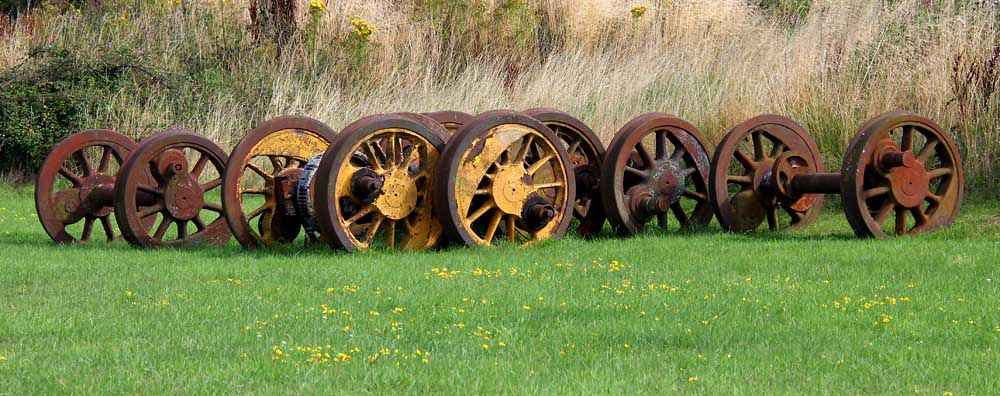This image depicts a serene, verdant field adorned with a mix of bright green, healthy grass and scattered yellow flowers. Dominating the foreground are approximately five sets of large, rustic metal wheels, each connected by a substantial metal bar. These wheels, weathered into a deep brown-red hue, evoke the industrial past, possibly part of an old plow or tractor from farmland history. Some of the wheel spokes are painted a striking yellow, contrasting with the overall aged appearance. Behind these relics, tall grasses, possibly wheat, provide a lush, blonde backdrop. The scenery is complemented by the trunks of distant trees, adding to the bucolic atmosphere of this outdoor tableau.